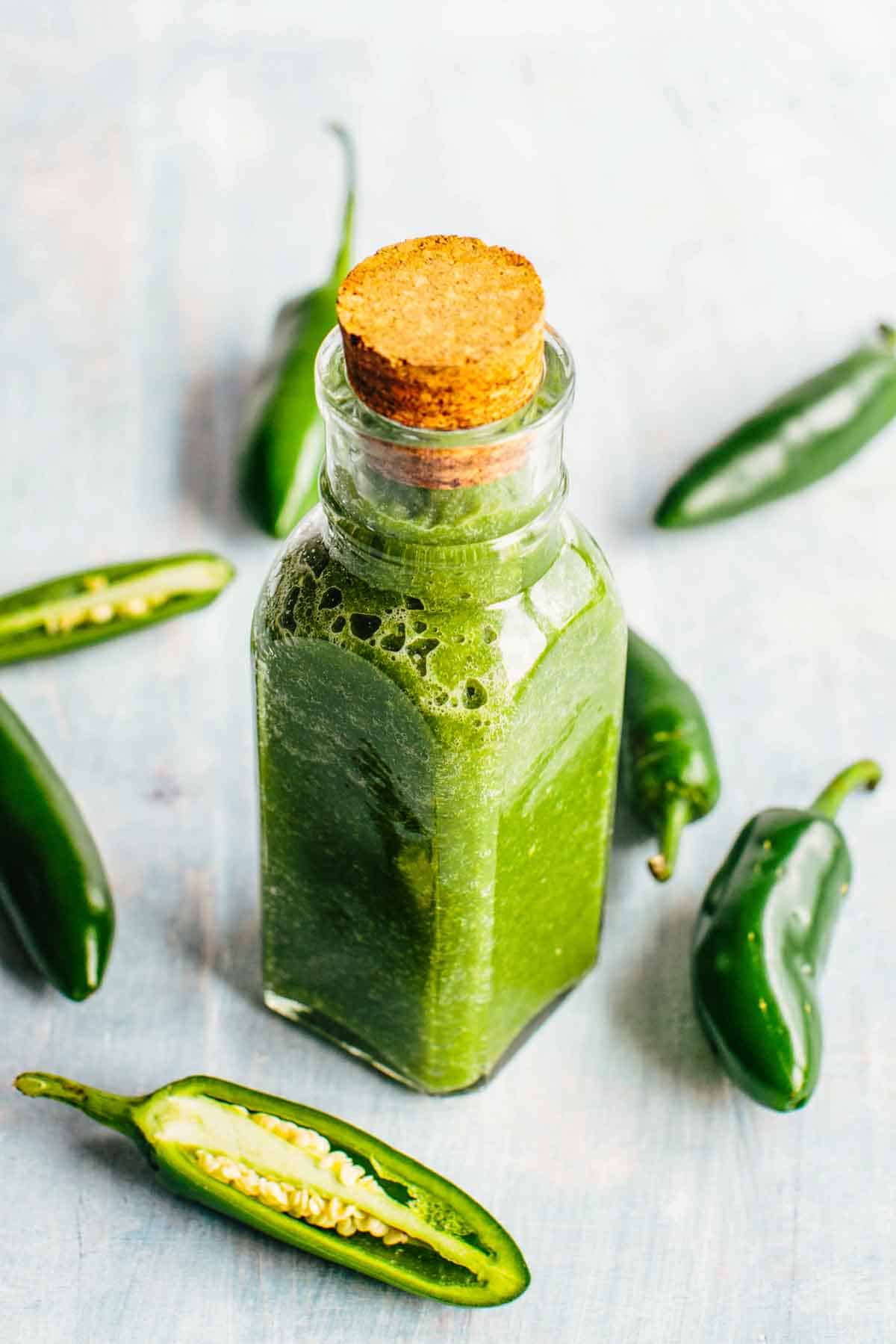This vibrant photograph captures a top-down view of an apothecary-style glass bottle filled with a bubbly, green jalapeño hot sauce, sealed with a cork stopper. The bottle, which is small and estimated to be around a couple of inches tall, is set against a dove grey wooden tabletop that subtly enhances the vividness of the green sauce. Surrounding the bottle, a variety of jalapeño peppers are artfully arranged; there are whole jalapeños in the distant background, with two on the left and three on the right. In the foreground, to the bottom-left, lies a sliced jalapeño showing its seeds, while another sliced half is placed midway up the image. Additional whole peppers decorate the scene, highlighting the fresh ingredients used for the sauce. This aesthetically pleasing composition emphasizes the harmony of green, yellow, tan, and soft grey tones, making the hot sauce look particularly tempting.